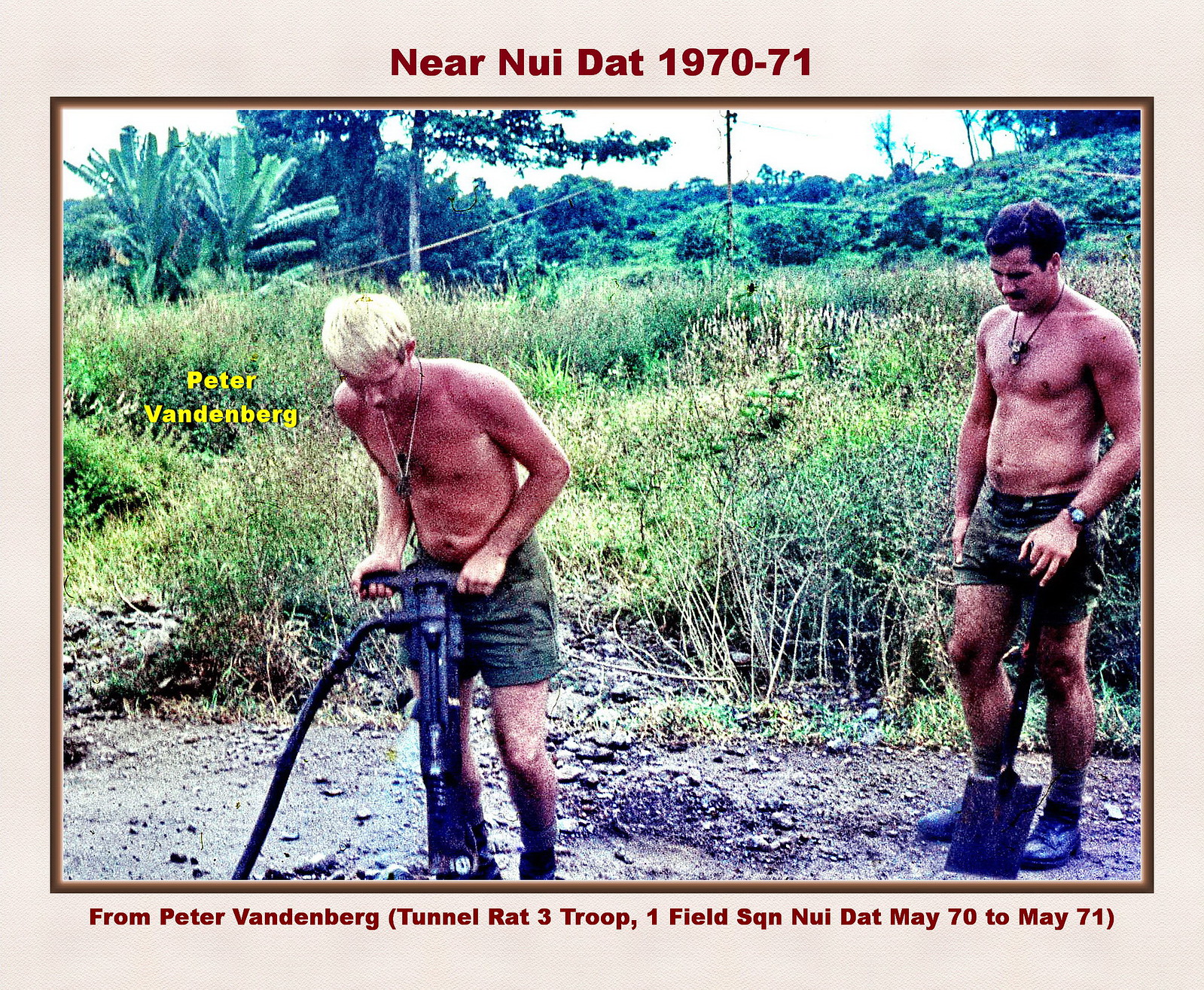This vintage photograph from the early 1970s, framed by a light tan border, captures two shirtless men working on a dirt pile amidst a backdrop of trees and bushes near Nui Dat, as highlighted by the brown text on the top and bottom borders. The top reads "Near Nui Dat 1970-71," while the bottom inscription states, "From Peter Vandenberg, Tunnel Rat 3 Troop 1 Field Squadron, Near Nui Dat May 1970-71." Both men are dressed in short green shorts, gray socks, and dark boots. The man on the right, a younger, muscular individual with black hair and a mustache, is adorned with a wristwatch on his left wrist and a necklace. He leans on a shovel, observing his companion. The man on the left, who is blonde and lean, also wears a necklace and is actively operating a jackhammer. The left side of the image features yellow text that reads "Peter Vandenberg." This detailed snapshot offers an evocative glimpse into the era and environment of these laborers, who appear robust and engrossed in their tasks against a verdant landscape.